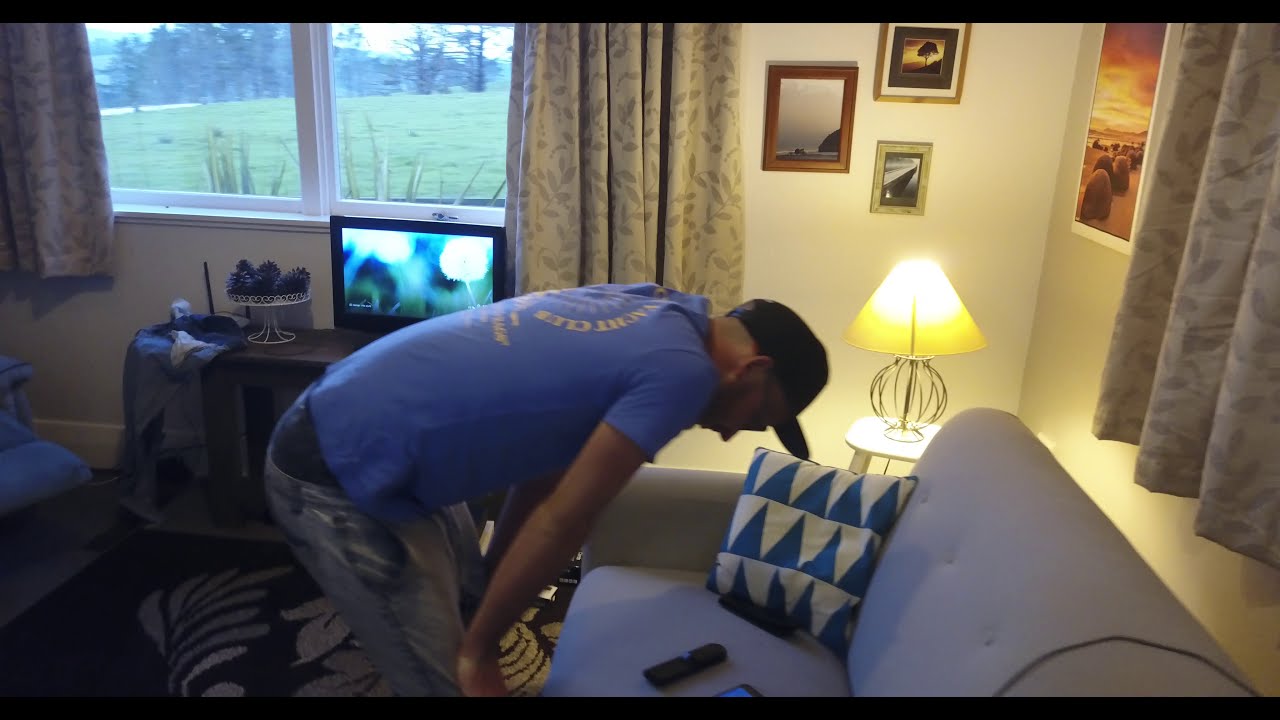This color photograph, taken from within a living room, captures a detailed and inviting scene. Centered prominently near the foreground, a man in a blue t-shirt with yellow lettering, jean shorts, and a black baseball cap is bent over a gray sofa. With his hands on his knees, he focuses intently on a cellphone lying on the couch beside a remote. The sofa is adorned with a white and blue geometric triangle pillow positioned in its corner. 

The living room features two windows with light gray curtains patterned with darker gray leaves, revealing a view of a large grassy area with trees under daylight. A small TV monitor sits on a wooden stand below one of the windows, accompanied by a decorative white wire basket containing pine cones. The walls, painted white, display several landscape photographs arranged neatly, with a trio of smaller frames on one wall and a larger vertical picture in the corner.

The room also contains a tufted blue and white floral rug, adding to its cozy ambiance. A glimpse of a blue cushioned chair can be seen to the left of the TV stand, further contributing to the room's comfortable and lived-in feel. The photograph is rich in detail, showcasing a blend of modern and homey elements that create a serene living space.